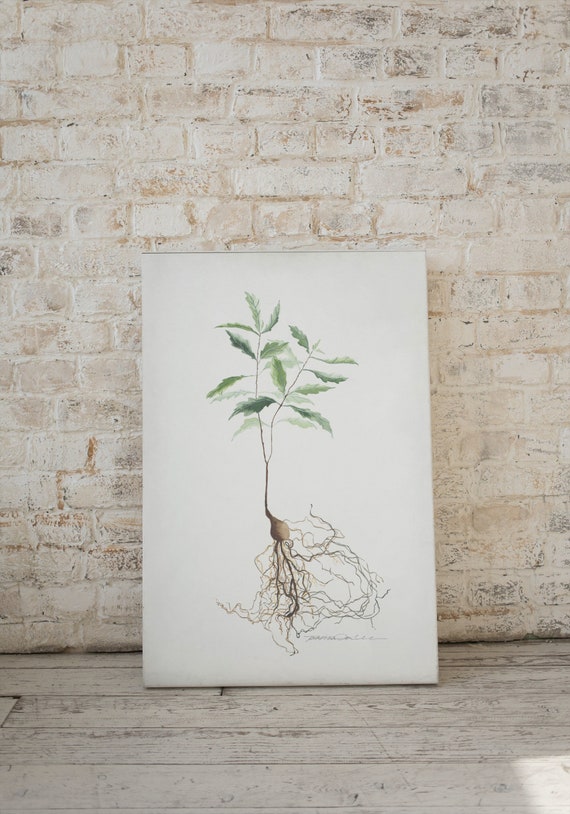The photograph showcases a detailed painting on a white canvas, depicting a small tree that has been uprooted, exposing its intricate roots. The tree, characterized by a relatively thin trunk and delicate branches, features approximately 20 green leaves. This artwork captures a tree seedling with two main branches emerging from the top, each adorned with a few leaves. Its roots, which are typically hidden beneath the soil, are prominently displayed against the stark white background of the canvas. This canvas leans against a white brick wall, which shows signs of age with patches of red and brown where the paint has worn away. The setting includes a weathered wooden floor painted white, with visible specks of brown mirroring the worn texture of the wall. A small, almost imperceptible artist's signature marks the painting, adding a final touch of authenticity to the composition.